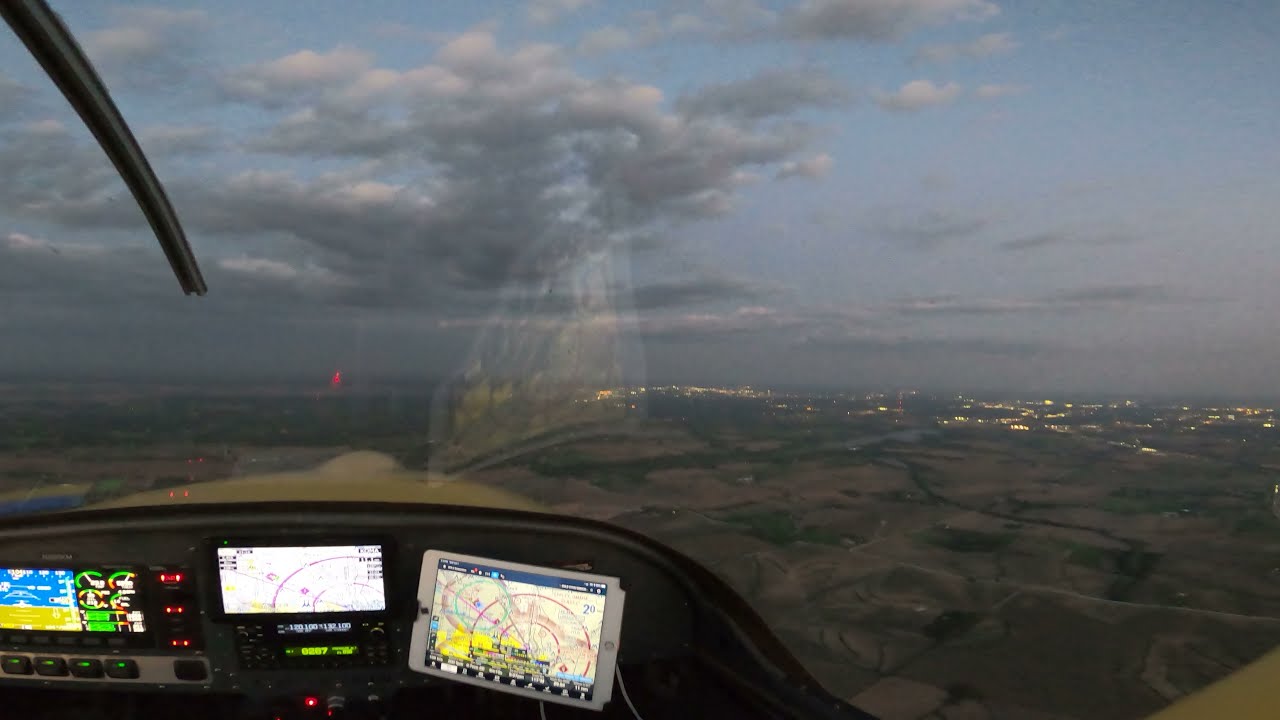The photograph captures the view from inside the cockpit of either a small airplane or helicopter. Prominently displayed on the dashboard are gauges and dials alongside three LCD screens, each showing various maps, radar images, and sonar readouts. In the lower left-hand corner, there are readouts possibly indicating speed and direction, along with some red indicator lights. Reflected in the windshield is part of the cockpit glass, and potentially the fuselage or tip of the aircraft, with something extending outward that could be a propeller blade. Outside the cockpit, the scene reveals a lush expanse of farmland below, interspersed with dirt patches. Further in the distance, beneath a partly cloudy sky casting a shadowed ambiance, the faint glow of city lights can be seen stretching across the horizon, transitioning the view from rural to urban.